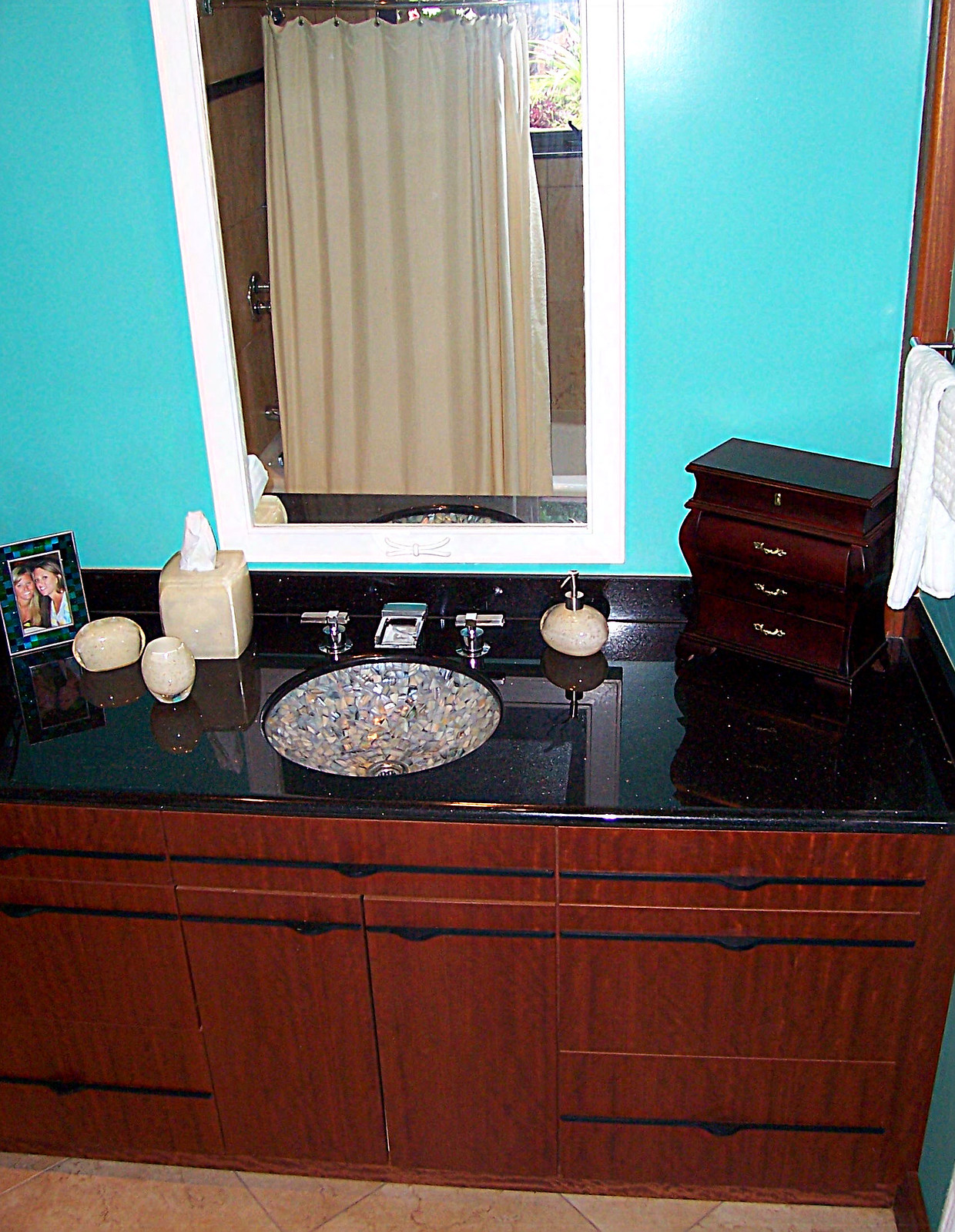The image captures an elegantly designed bathroom, the centerpiece of which is a striking mosaic sink. This sink, adorned with a flashy, shiny mosaic of various colors, immediately draws attention due to its vibrant contrast with the rest of the bathroom’s decor. In stark comparison, the sink's taps are simple bars projecting outward, embodying a minimalist design. Above the sink, a wall-mounted mirror reflects a beige shower curtain, which dominates the background.

The bathroom walls are painted a vivid ocean blue, creating a lively atmosphere and providing a bold contrast to other elements in the room. Situated directly beneath the sink, a set of dark brown, well-furnished wooden cabinets offer a robust foundation, their deep tone adding a touch of sophistication. Complementing these cabinets is a small chest of drawers placed on top, matching in color and finish, enhancing the cohesive dark wood theme within this vibrant and well-appointed bathroom.